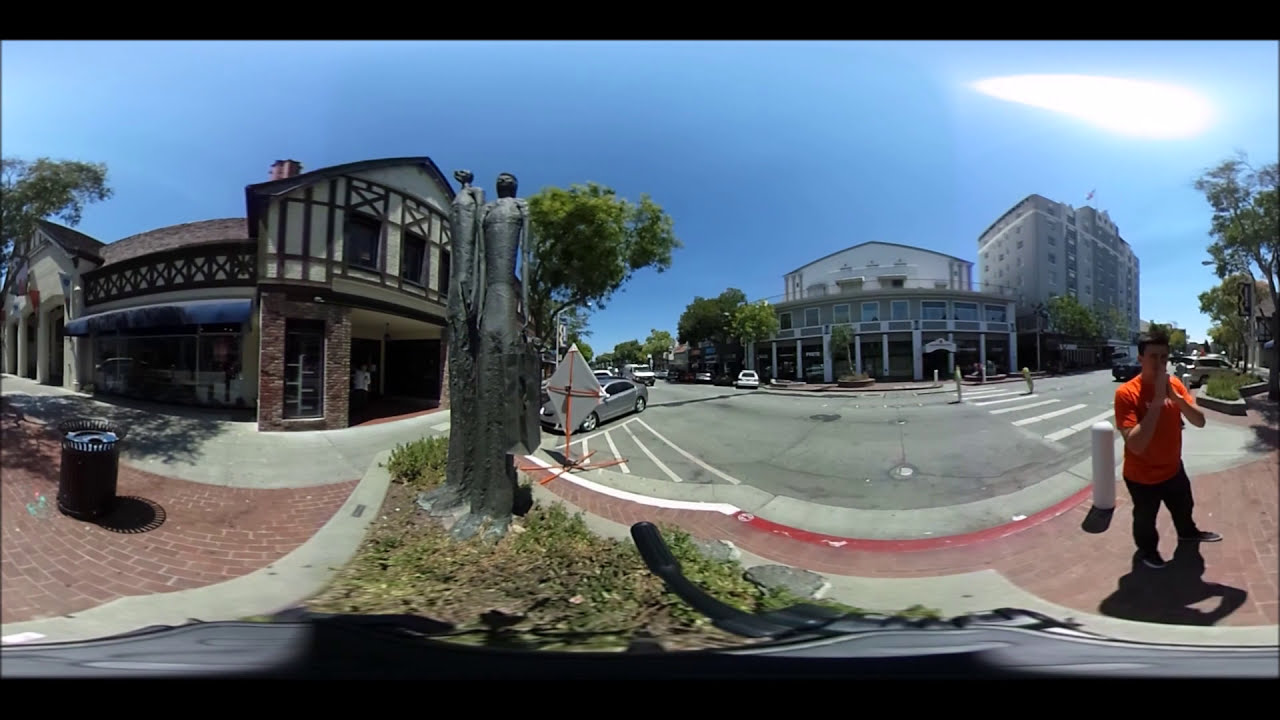The image captures a 360-degree panorama of a European townscape, characterized by a distinctively warped and curvy perspective, imparting an almost surreal quality to the scene. At the bottom, a narrow strip reveals a possible bicycle helmet, hinting at the photographer’s method of traversing the area. To the left, a red brick courtyard transitions into a cement walkway, leading up to a traditional building with brown brick and white walls, accentuated by wooden framing reminiscent of German Fachwerk architecture. 

Center-stage within a grassy median stands a pair of elongated, metallic humanoid statues, their exaggerated tall forms casting an intriguing silhouette against the setting. To their right, a white crosswalk marks the beginning of an open street, flanked by cars parked on the left side and lined with modern, gray and white buildings on the far side, towering like apartment or hotel complexes. Extending to the far right corner stands a man, likely in his 20s, wearing an orange t-shirt. Above this urban tableau, a vibrant blue sky stretches out, with the sun elongated in the upper right corner due to the panoramic effect. The overall image is framed by thin black bands at the top and bottom, adding to the distinct visual presentation.